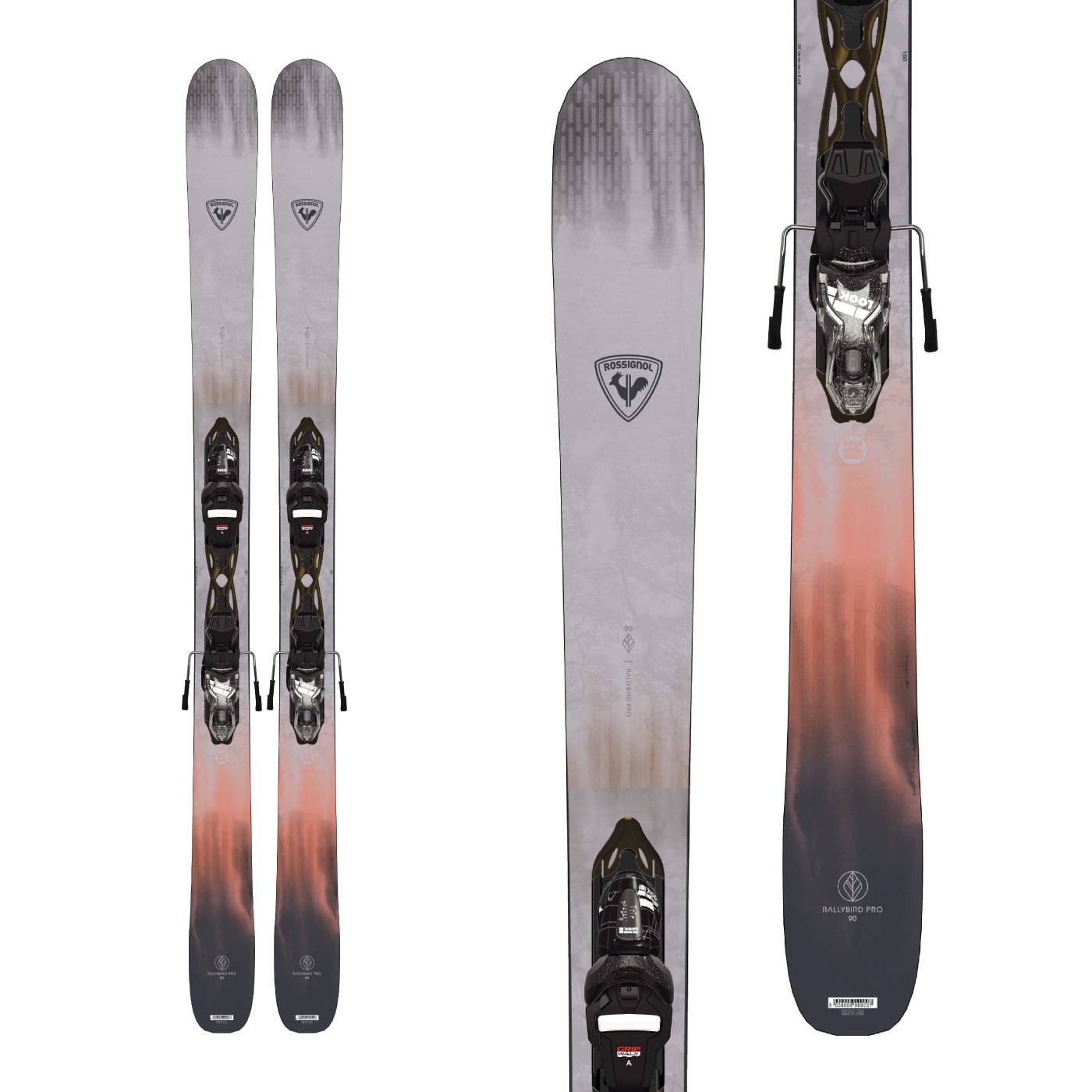This image appears to be a detailed advertisement photograph showcasing a pair of Rossignol skis. The background is entirely white without any borders, emphasizing the skis. On the left side of the image, there are two identical skis displayed parallel to each other, showing them from top to bottom. The skis feature a color scheme that includes gray, orange, pink, black, and white. The top part of the skis has a smeared black design over a white base, with a triangle logo showing a rooster and the brand name "Rossignol." The middle section, where the black bindings are located, is prominently displayed. Additionally, there are some wispy orange accents towards the bottom, which culminates in a blend of gray and pink colors.

On the right side of the image, there's a zoomed-in view focusing on different parts of the skis: one close-up of the front end, showing the logo and part of the binding, and another of the back section highlighting more binding details. This comprehensive display allows viewers to appreciate the full design and specific features of the skis, including the branding and intricate color patterns, making it apparent that this photograph aims to meticulously present the product from multiple perspectives.